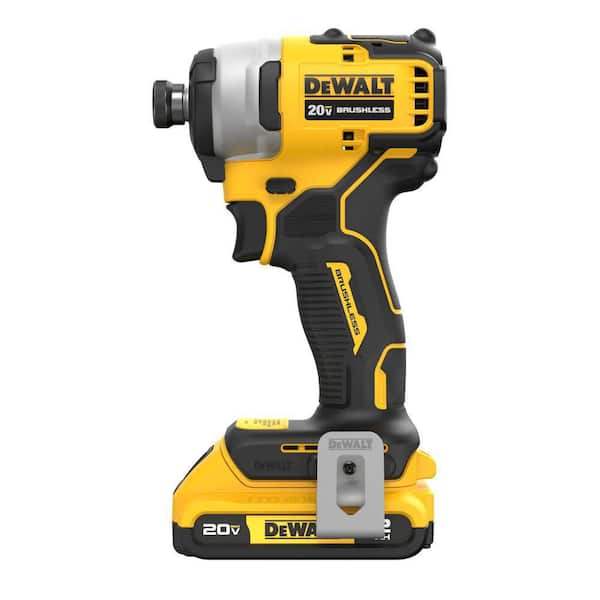This image showcases a DeWalt 20V BRUSHLESS handheld power tool, prominently featuring the brand's classic black and yellow color scheme with a mix of gray and silver accents. The tool, which appears to be a drill or compact driver, exhibits a gun-like shape, with its functional end positioned to the left of the viewer. The front section of the tool where attachments like drill bits or brushes can be connected is black, while the body bears the "DEWALT 20V BRUSHLESS" branding in multiple places—front, handle, and bottom. The tool's handle also includes a silver clip for added versatility. The device is displayed as just the base unit, mounted on its 20V battery for stability and balance in usage, with no extra accessories or bits attached.